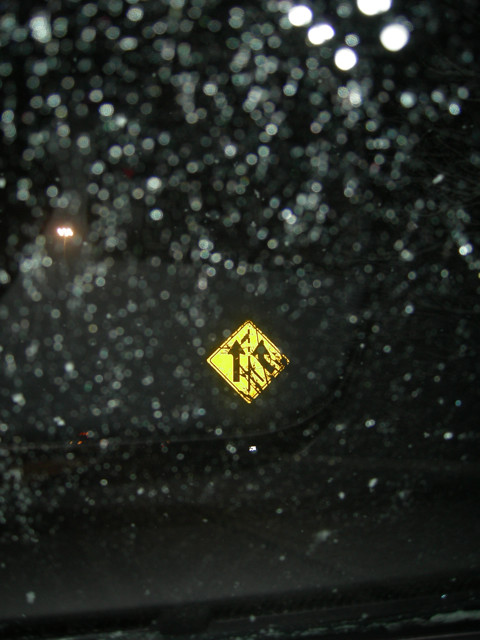The photograph captures a scene through a vehicle window heavily dotted with droplets of water, likely from rain or ice. The slightly obscured view reveals the dark interior of the car, including a black dashboard at the bottom of the image. In the distance, amidst the darkness, a single tall lamppost with multiple bulbs can be faintly seen, casting light that reflects off the droplets.

The focal point of the image is a yellow, diamond-shaped roadside sign visible through the rearview mirror. This sign, centered in the middle of the photograph, features two black arrows separated by a vertical black line: the left arrow points straight up, indicating a forward direction, while the right arrow curves upward to the left, suggesting a merging lane. The scene feels somewhat ethereal with the numerous white orbs created by the light reflecting off the water droplets, enhancing the overall sense of a rainy or icy night.